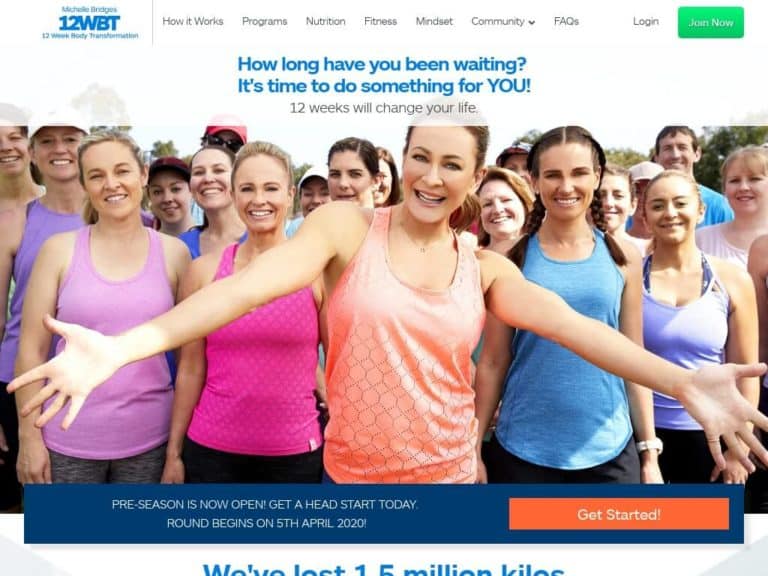The screenshot depicts a webpage from the official site of Michelle Bridges' 12 Week Body Transformation (12WBT) program. In the top-left corner, the logo reads "Michelle Bridges 12WBT" in blue text. Navigation tabs with grey font are aligned across the top of the white background, labeled: "How It Works," "Programs," "Nutrition," "Fitness," "Mindset," and "Community." The "Community" tab features a downward arrow indicating a drop-down menu, followed by additional links including "FAQ," "Log In," and a prominent green "Join Now" button.

Central to the page is a motivational headline in blue font proclaiming, "How long have you been waiting? It's time to do something for YOU!" with "YOU!" in all caps for emphasis. Beneath this, a subheading in light grey font declares, "12 weeks will change your life." 

The middle section showcases an inspiring image of various women, primarily aged 30 and above, dressed in workout gear with one man visible in the background to the right. At the bottom, a blue banner announces, "Pre-season is open now. Get a head start today. Round begins on 5th April 2020." Adjacent to this is an orange call-to-action button with white text that reads, "Get Started."

Though partially cut off, additional text hints at the program's success, stating that participants have collectively "lost 1.5 million kilos." The use of kilograms suggests that the website likely caters to a European or British audience.